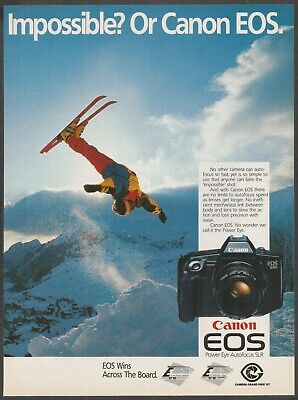This full-page advertisement from what is likely a periodical or magazine features a Canon EOS single-lens reflex (SLR) camera. The advertisement's focal point is a vivid, high-action photograph of a skier in mid-flight, performing a backflip off a snowy bank. The skier is spectacularly suspended in the air with his head below his skis, legs extended forward roughly at a 45-degree angle, and arms fully extended, indicating he is about a third of the way through the backflip. He's dressed in multicolored ski gear, including a yellow, orange, and blue torso, red pants, and red and yellow skis. A bright blue sky with the sun and wispy clouds, along with a sweeping, snow-covered mountainous landscape, serves as the backdrop.

Situated prominently at the top of the advertisement in large white font, the text reads: "Impossible? Or Canon EOS." An inset within the ad displays the Canon EOS camera itself. The camera appears sturdy and professional, characterized by a black DSLR body, a sizable circular lens, and a grip on the right-hand side. Below the camera image, there is the Canon logo in red followed by "EOS" in large black font, all set within a white rectangular background.

One distinctive design element is an overlay near the camera, presenting a white rectangular section at the bottom of the ad with text proclaiming, "EOS wins across the board." This section also contains three logos, likely representing awards that the Canon EOS camera has received, although the specific text and details of these logos remain too small to discern.